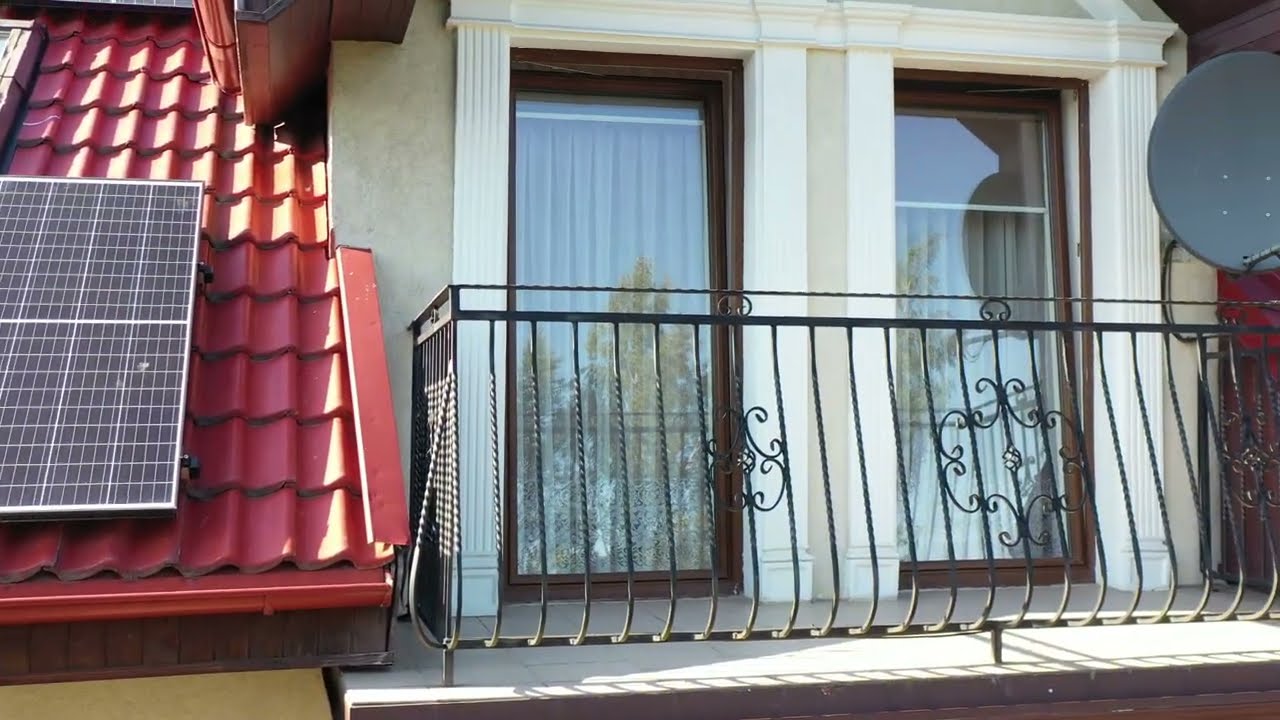The image depicts the top floor of a house with intricate architectural details and outdoor amenities. The focal point is the white facade featuring two large glass windows adorned with elaborate white molding. These windows open out onto a small balcony enclosed by an elegant black wrought iron railing, which is decorated with decorative fleur-de-lis patterns. A gray satellite dish is mounted on this railing, and the balcony offers a view of the surroundings, including a reflection of eucalyptus trees. Adjacent to the balcony, the roof is covered with terracotta-red tiles and features a mounted solar panel composed of eight smaller panels. The roof has red guttering, enhancing its detailed finish. The day is sunny with clear blue skies, contributing to the sharpness and clarity of the image.